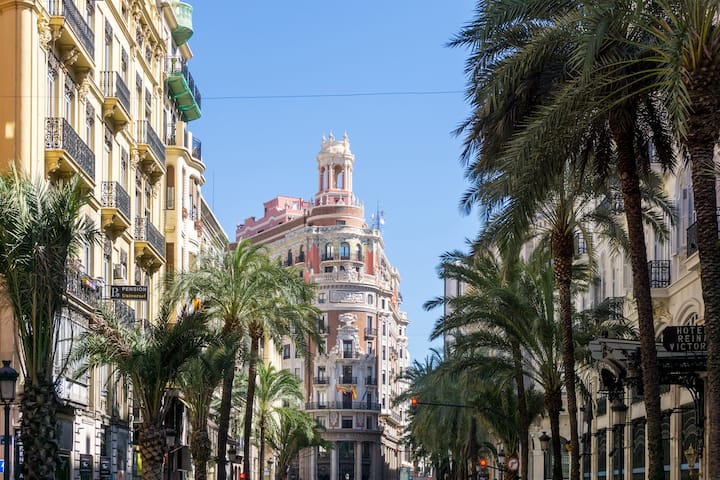This image captures a vibrant city street flanked by palm trees and large, ornate buildings. At the end of the long roadway stands a very tall and elaborate pink and white building, distinguished by its triangular shape and a splendid tower featuring arched windows and a white roof. The building's intricate design is crowned with a cupola, offering views of the city. On the left side of the scene, there's a notable building adorned with green-painted and wrought iron balconies, while a yellowish building on the right displays more ornate balconies and a sign that partially reads "Hotel Reina Victor." Together, these details suggest a stylish, potentially Spanish cityscape, bustling with architectural charm and tropical greenery.